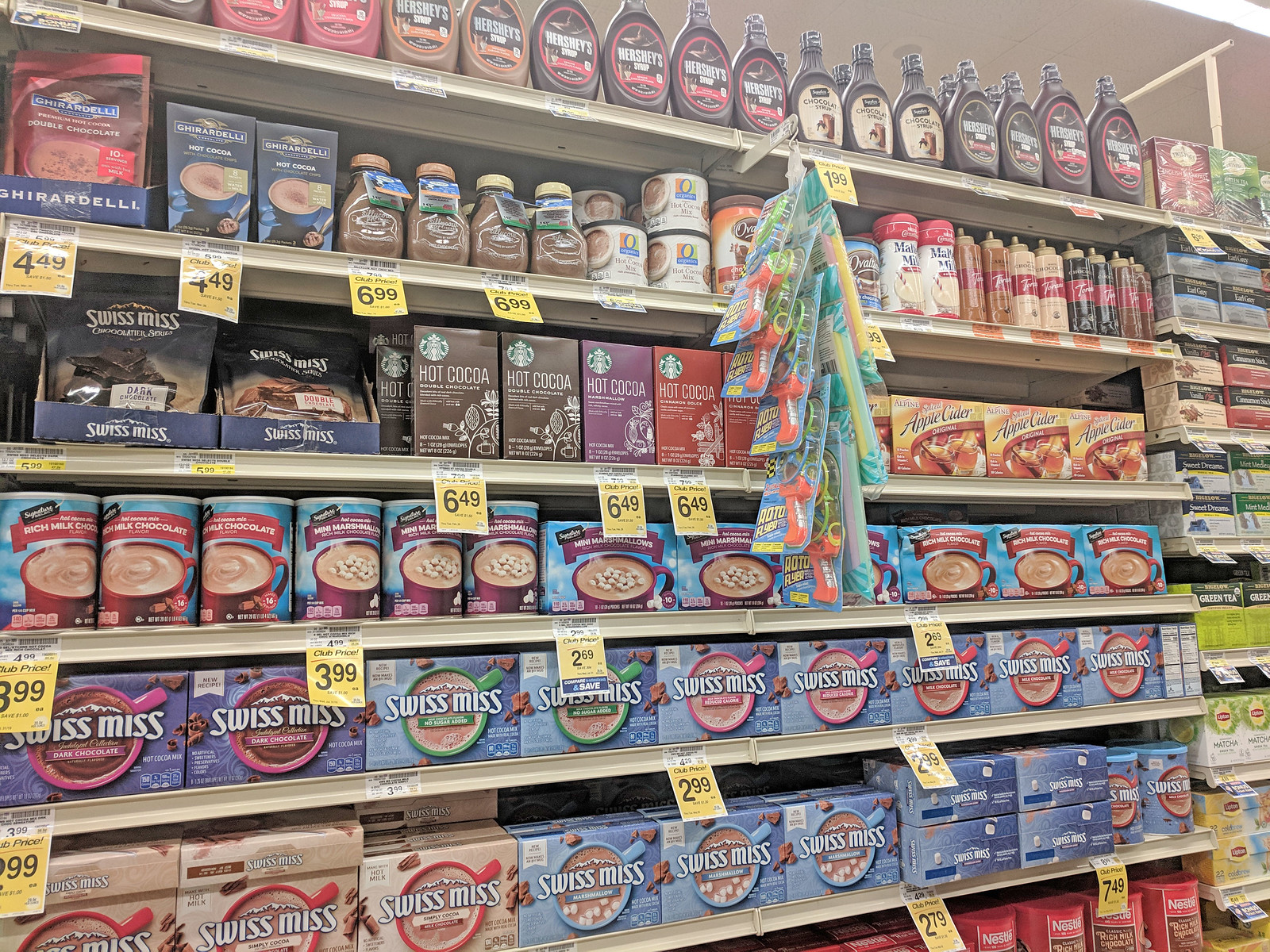This image depicts a well-stocked grocery store aisle with seven visible shelves filled with a variety of hot chocolate, tea, syrups, and related products. The bottom two rows prominently feature an assortment of Swiss Miss hot chocolate boxes, followed by store brand hot chocolate. Above these, mid-shelves display Starbucks hot chocolate, Swiss Miss chocolate bark, and boxes of apple cider. Moving upwards, you can see a selection of caramel and chocolate syrups on the second-to-the-top row. At the very top, a variety of Hershey's syrup bottles, including strawberry, caramel, and chocolate, are neatly arranged. Yellow price tags indicating various prices such as $6.99, $3.99, $2.99, and $1.99 are visible on every row, enhancing the detail and reality of the shopping scene.